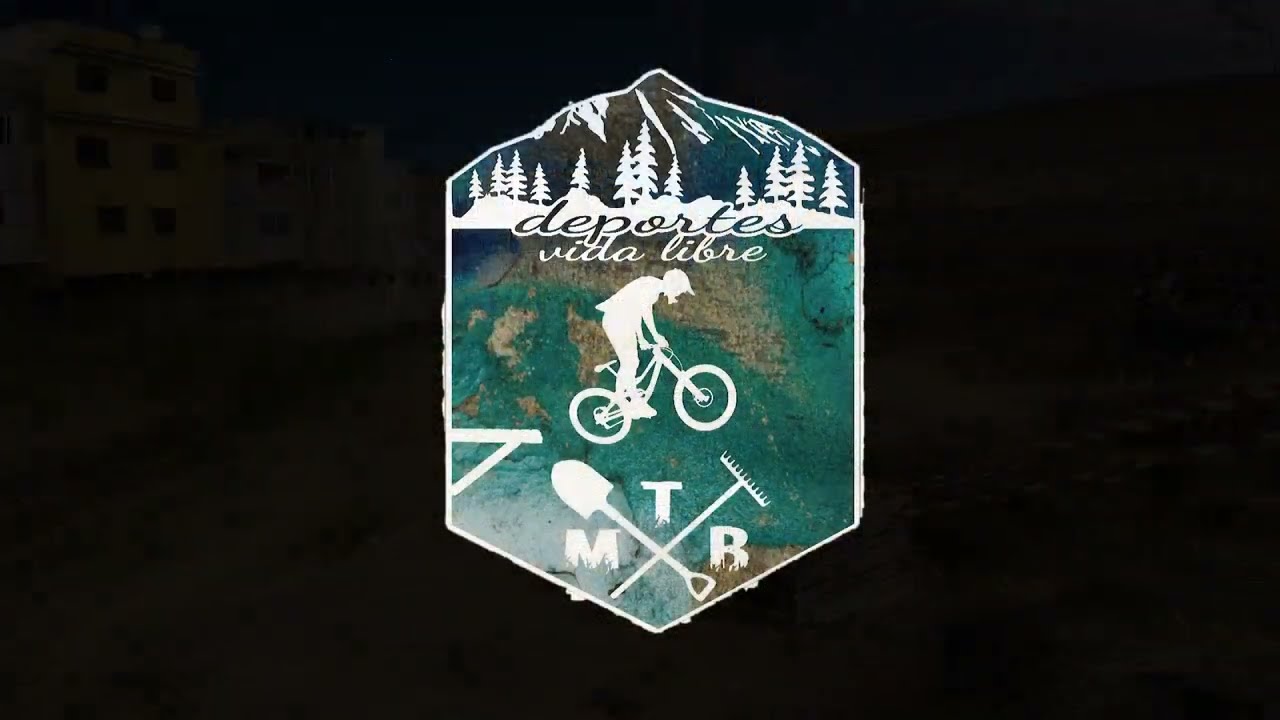The image features a central logo set against an almost black, shadowy background that's hard to distinguish. The background seems to depict a very dark scene of a town with faint outlines of buildings, trails, and possibly a body of water. The central logo is a hexagon shape with detailed, colorful elements. 

At the top of the hexagon, there is a cartoon depiction of a mountain – its right side green and left side brown – with white pine trees standing in front. Below this, the background transitions into a map-like terrain with green and brown elements. Dominating the center of the hexagon is a white silhouette of a person performing a BMX jump off a ramp, standing on the pedals and wearing a helmet. 

Directly below the BMX rider, a shovel and rake are crossed to form an 'X', with the letters "MTB" in white capitals prominently situated around the tools. The words "Deportes Vida Libre" are displayed within the hexagon, likely indicating the name of an outdoor or adventure company focused possibly on mountain biking, as suggested by the imagery.